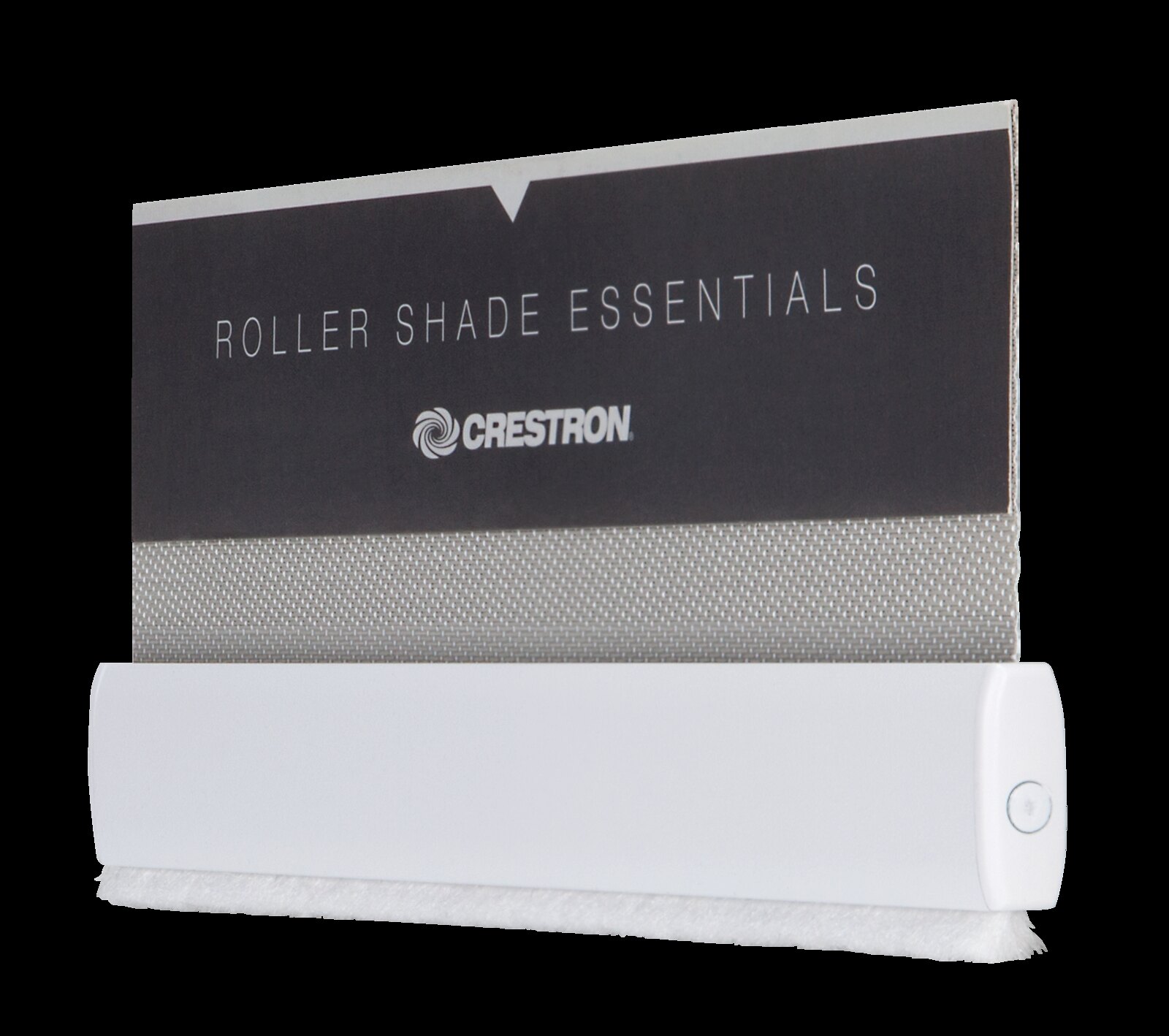The image features a sign with a black border, which is not perfectly rectangular. At the top of the sign, in a centered, light blue, thin capital letter font, it reads "Roller Shade Essentials." Below this text, there is a swirl-shaped icon resembling a flower, situated to the left of the word "Crestron," which is written in a thicker, bold white capital font. The middle section of the sign is a lighter gray, filled with intersecting vertical and horizontal stripes, creating a pattern of small white dots. Beneath this area, there is a depiction of a white roller apparatus, suggesting the bottom part of a rolled-up item, possibly a shade. Below the apparatus, a white shade material is shown hanging down. The whole composition appears to be set against a dark gray background, making the text and design elements stand out.